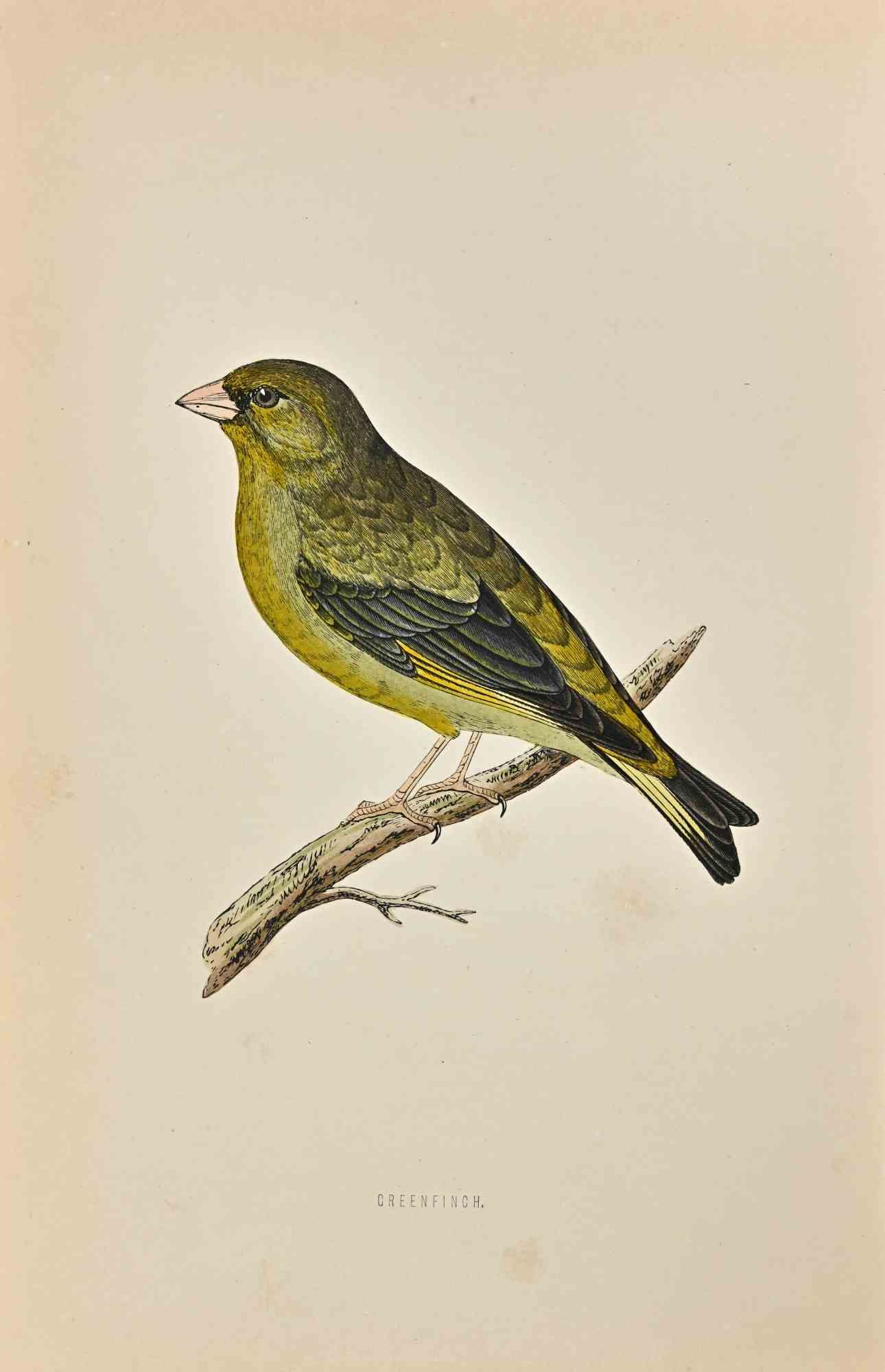The image is an old, weathered page from a textbook or pamphlet, featuring a detailed illustration of a Greenfinch. The bird, depicted in a realistic yet slightly cartoonish style, stands perched on a slender, light brown branch. The Greenfinch boasts a vibrant green plumage with feathers tinged in shades of yellow and gray. Its short, wide beak is prominently visible, and the tips of its wings and tail feathers are darker, almost black, forming a distinctive heart shape. The background is a neutral grey, enhancing the vintage feel of the illustration. Small text at the bottom of the page labels the bird simply as "Green Finch."